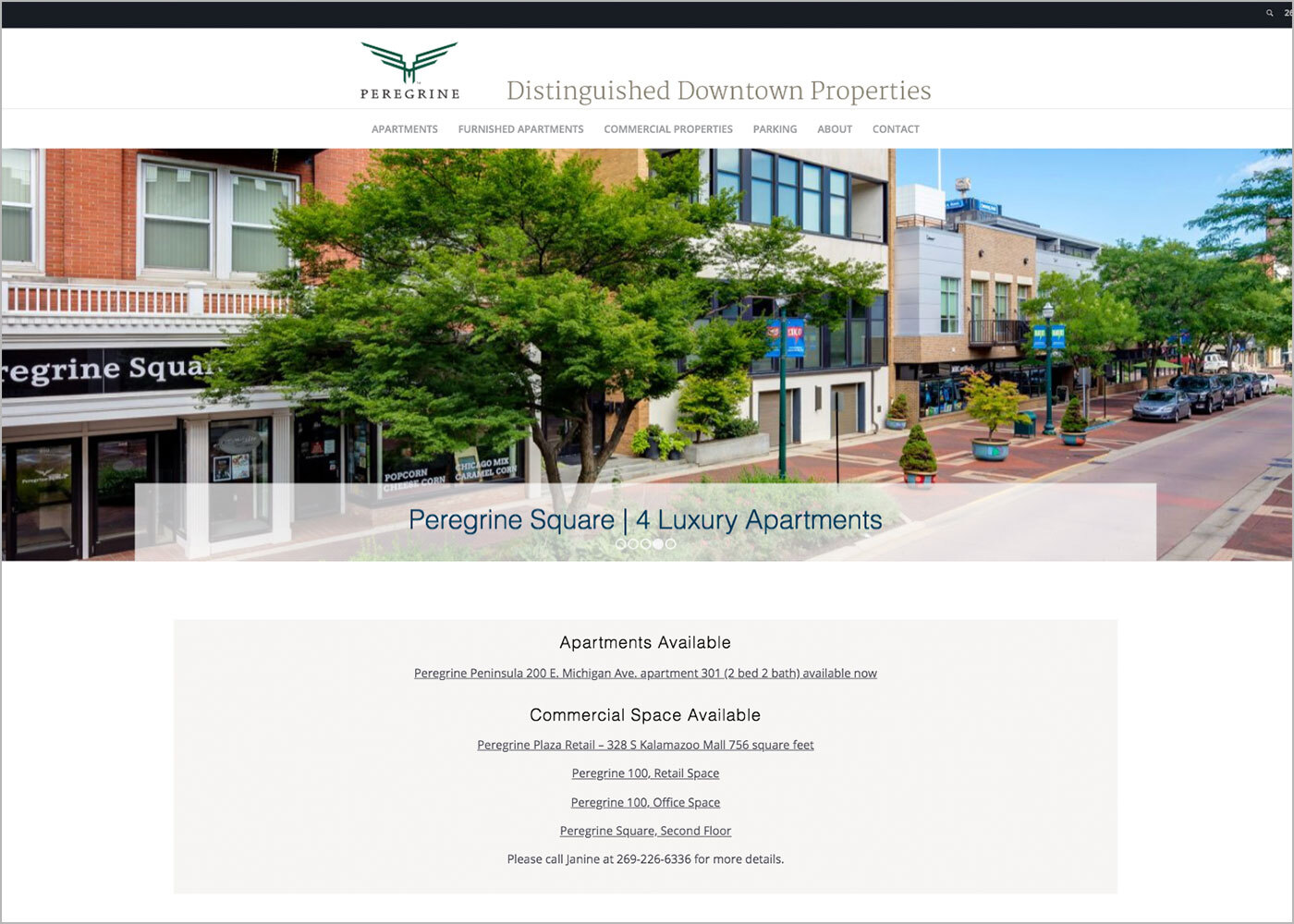This website image showcases Peregrine Properties, known for their distinguished downtown apartments and commercial spaces. At the top, there is a sleek black border, immediately followed by a crisp white section featuring Peregrine's elegant green logo, which depicts a bird with spread wings formed by three lines. The logo is accompanied by the text "Peregrine, P-E-R-E-G-R-I-N-E," and below it reads "Distinguished Downtown Properties" with navigation options for Apartments, Furnished Apartments, Commercial Properties, Parking, About, and Contact.

The main image highlights a picturesque urban scene with apartment buildings situated above charming shops. The area, known as Peregrine Square, is adorned with lush green foliage and street-side trees, while cars line the road, emphasizing a lively downtown ambiance. Key information displayed includes:

**Peregrine Square**:
- Four luxury apartments available now.
- **Peregrine Peninsula**, at 200 East Michigan Avenue, Apartment 301:
  - Two-bedroom, two-bathroom
  - Available immediately

**Commercial Spaces**:
- **Peregrine Plaza Retail**, 328 Kalamazoo Mall:
  - 750 square feet
- **Peregrine 100 Retail Space**
- **Peregrine 100 Office Space**
- **Peregrine Square second floor**

For more details, please contact Janine at 269-226-6336.